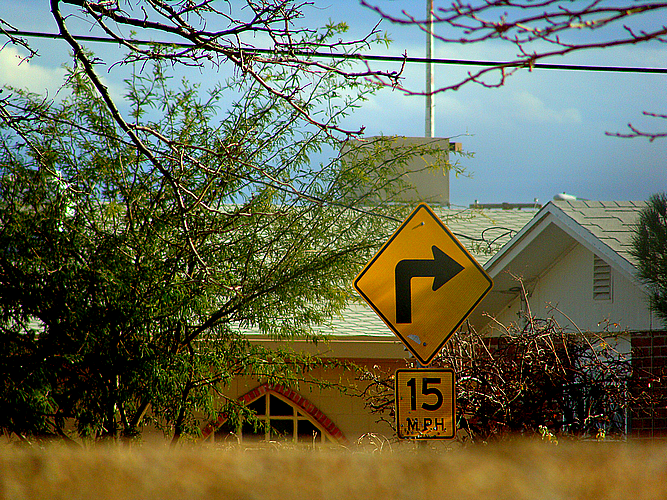The image depicts a yellow, diamond-shaped speed sign indicating a sharp turn to the right. Below the sign is a square placard stating a speed limit of 15 miles per hour. The sign is positioned in front of a residential building, partially obscured by a tan-colored privacy wall. The house features a large window with brick accents and window dividers, and its roof is adorned with a sizable chimney. Additionally, there is a vertical pole situated behind the chimney, with an electrical wire running in close proximity to the house. Trees are visible in front of the building, adding a touch of greenery to the scene.